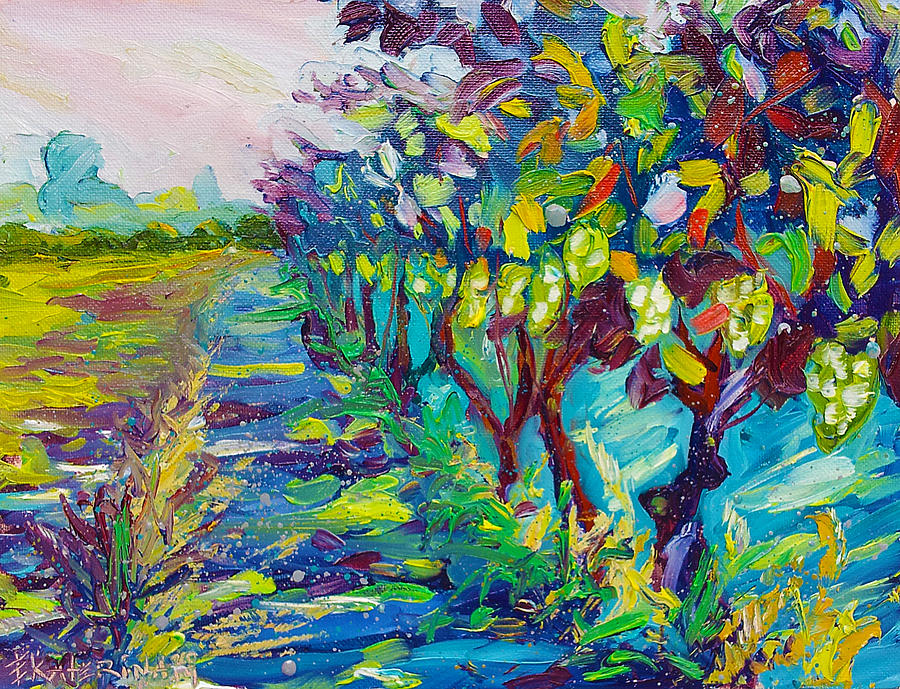This impressionist painting, possibly in oil or acrylic on canvas, depicts a vibrant daytime outdoor scene characterized by a dynamic explosion of colors and textures. The right side of the composition features several short trees adorned with a multitude of flowers in colors such as white, brown, yellow, red, green, purple, and dark blue. These trees, though small in height, transition into heavily textured, thick strokes of paint that capture the essence of blooming flora. The central part of the image has a subtle mix of blue and green hues, leading towards the background where a blue sky with little pink clouds meets the vibrant landscape. To the left, the ground is initially grassy, merging seamlessly into a sea of multi-colored flowers—blue, light green, yellow, red, pink, purple—that stretch across to the right. The background also shows more vibrant pink skies. The scene includes a small moat or water body running parallel to the tree line. The artist's signature, "Katerina," is subtly blended into the sea of flowers in the lower left corner, along with a symbol and a print number "260." This intricate image captures the essence of a colorful, impressionistic landscape filled with boundless natural beauty.